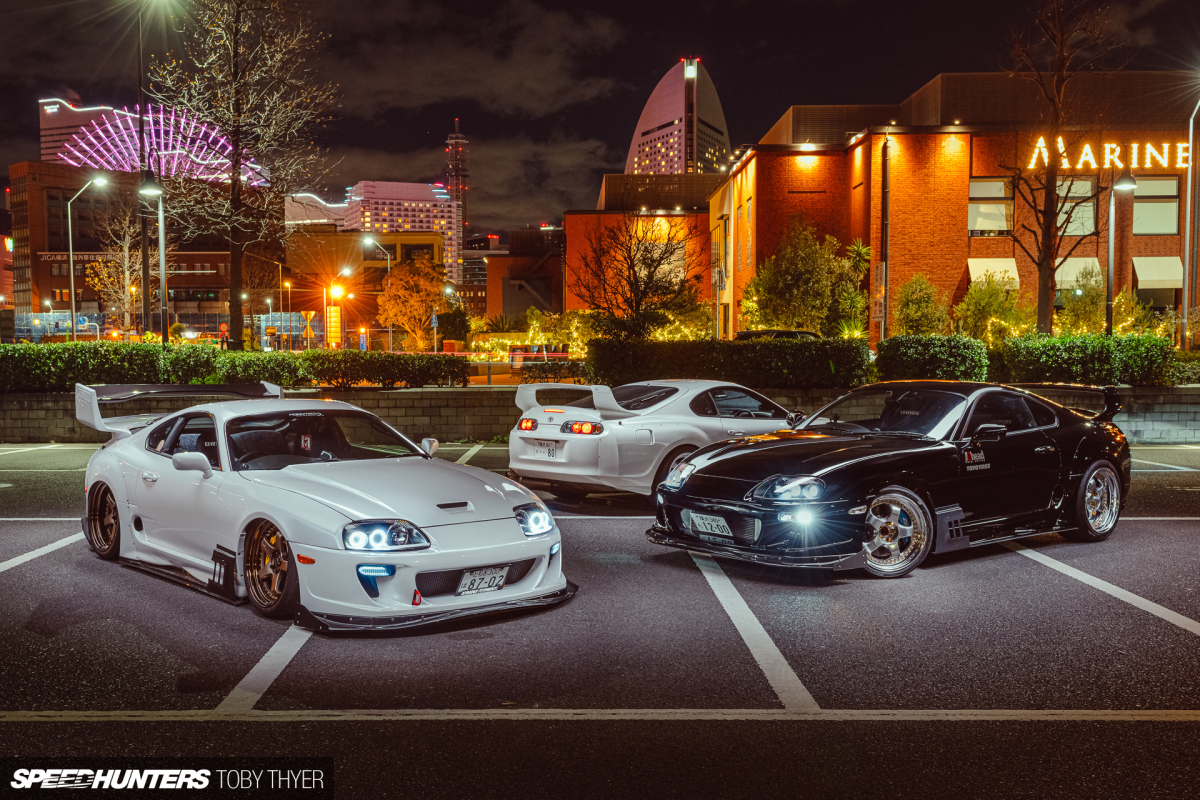The image showcases three sleek sports cars parked in a lot, against the backdrop of multiple buildings, including hotels. Two of the cars are white; the third, positioned at the front, is black and resembles a Porsche. The scene is set at night, illuminated by street lights that highlight the cars' sporty and new appearance. The buildings in the background include a hotel with "Marine" written in white letters, and another structure glowing with a neon purple light. The entire setup, which might be 3D generated or from a video game, creates an uncanny valley effect. The bottom of the image features the text "Speed Hunters" alongside a logo and the name "Toby Fire," suggesting it might be part of a digital artwork or gaming interface. The visual elements include a mix of whites, blues, greens, blacks, yellows, reds, and neons. The overall scene, rich in detail, yet ambiguous in its realism, sets a vibrant but enigmatic urban mood.